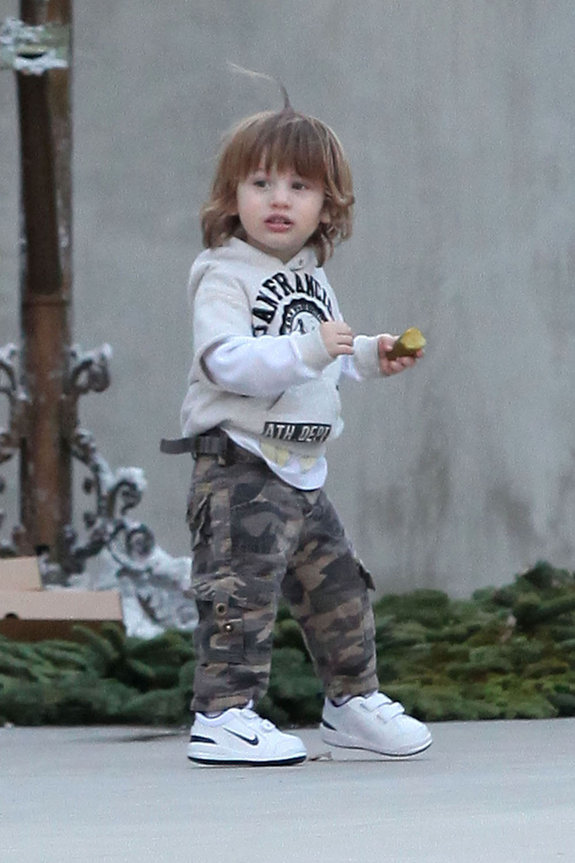This is a detailed photograph of a young boy with shoulder-length brown hair and bangs, captured outdoors on a concrete or asphalt surface. He is dressed in a white, long-sleeve hooded sweatshirt that extends to his wrists. The sweatshirt features the word "San Francisco" in a black arch with a circular black emblem that is somewhat indistinct beneath it. Around the stomach area, there's a black bar with white writing that reads "A-T-H D-E-P-T," shorthand for "Athletic Department." He pairs this with long gray camouflage pants. On his feet, he wears white Nike velcro sneakers, which have a black Nike swoosh on the visible side, black soles, and a distinctive white line on the back heel.

In his left hand, the boy holds a piece of a donut, suggesting he is in the middle of eating. He is facing to the right but glances back over his right shoulder, directing his eyes towards the camera. The background reveals a gray stone wall lined with low green bushes at its base. Additionally, a decorated iron post, painted white at the bottom, is visible to the left of the boy.